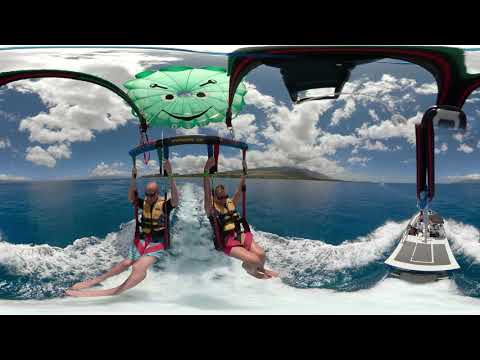In this photograph of a parasailing adventure, two people are suspended in harnesses just above the shimmering blue water, attached to a boat visible on the right side of the image. The man on the left wears black goggles, a black t-shirt, blue shorts, and a yellow and black life jacket. He is bald and grips the harness straps with both hands. The woman on the right has blonde hair, black goggles, pink shorts, and an identical life jacket. They are both connected to a black bar and their feet are just above the water’s surface, causing small ripples as they skim along. The green parachute above them features a cartoon-style smiley face in black and white. The entire setup is tethered to the boat by black and red straps. The scene is set against a backdrop of bright blue sky with large fluffy clouds and a small green and brown island near the center of the image. Overall, the image captures a vibrant and joyful moment of parasailing on a sunny day.